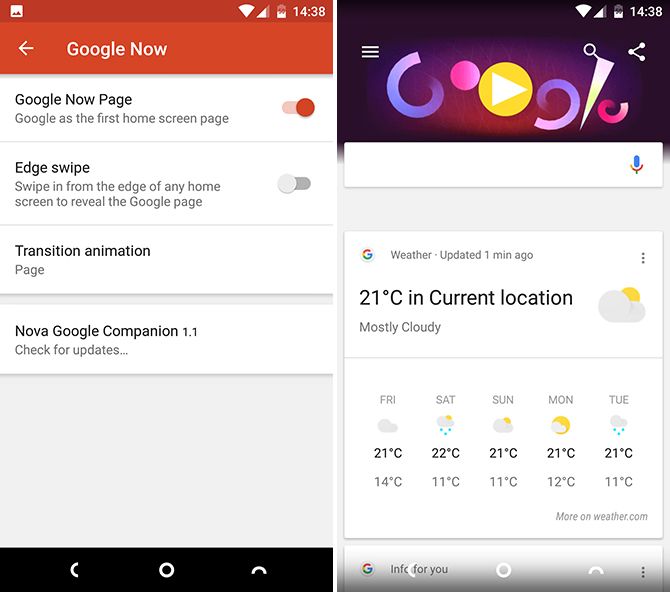This detailed caption describes an image featuring two smartphone screenshots placed side by side:

---

In the left screenshot, the top header is a maroon color, displaying the time as 14:38 in a 24-hour format. Beneath that, a slightly lighter brick-red header features "Google Now" in white font with a left-pointing arrow. The main section has a white background, presenting various options from top to bottom: 

1. **Google Now Page** - Selected, indicated by a red button on the right.
2. **Google as the First Home Screen Page** - Also selected.
3. **Edge Swipe** - Not selected, marked by a gray button.
4. **Transition Animation**
5. **Nova Google Companion 1.1**

The right screenshot shows consistency in the top display with the same time and battery indicator. Here, we see an interesting Google logo with a blue background and red center. The word "Google" is written in whimsical colors. Below it, a familiar search box is present. Underneath is a weather widget indicating 21 degrees Celsius at the current location. The forecast for Friday through Tuesday is displayed below, including the highs and lows for each day, along with icons depicting rain, sunshine, or clouds.